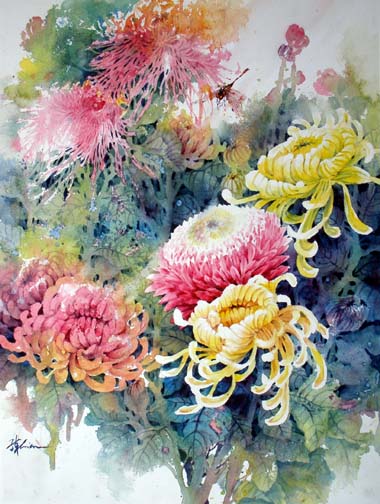This vibrant and striking painting showcases a mystical bouquet of flowers, with a predominant color scheme of pinkish magenta and yellow. The flowers, featuring spherical shapes made of curved, thin petals—each flower boasting over a hundred petals—float gracefully above a green base and stalks. The leaves and stalks exhibit a mesmerizing blend of blues, purples, and darker greens. While primarily pink and yellow flowers take center stage, hints of smaller red flowers in the background add to the composition's rich color palette. The image, relatively abstract yet detailed, is signed in the bottom left corner, grounding the otherworldly scene with an authentic, artistic touch.